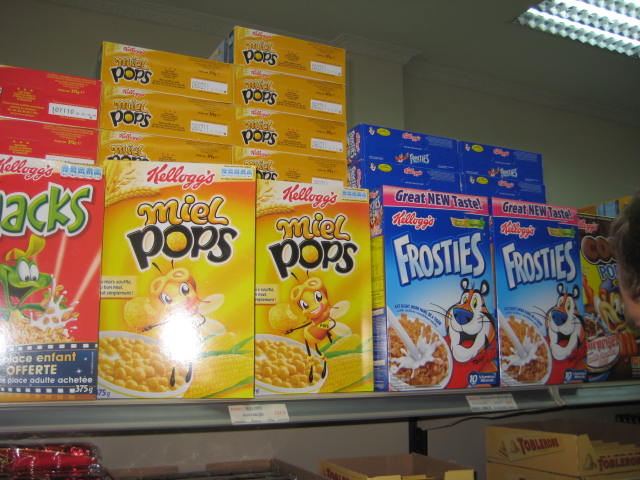This photograph captures a store shelf laden with various Kellogg's cereal boxes, showcasing impeccable product arrangement and vibrant packaging. On the top shelf to the left is a red box of Kellogg's Apple Jacks, partially obscured but identifiable by its green lettering and cheerful green frog mascot. Adjacent to this are two boxes of Kellogg's Miel Pops, characterized by a bright yellow and orange design, featuring a happy bee hovering above a bowl of honey-coated pops and a corn on the cob imagery. Further right, two blue boxes of Kellogg's Frosties proudly display Tony the Tiger, enthusiastically presenting a bowl of cereal with milk pouring into it and a red banner announcing a new great taste. Behind these, additional boxes are stacked, forming a visual back stock. Along the bottom shelf, noticeable Toblerone packaging and shiny red wrappers add a splash of variety. Just within the frame on the right, a person's hair, chin, and cheek are visible, as well as a brown and yellow box featuring a bear mascot likely representing a cocoa-flavored cereal. Small white price tags line the bottom shelf, indicating the prices of the cereals. The photograph is slightly dark, adding a moody, realistic atmosphere to this snapshot of grocery store life.